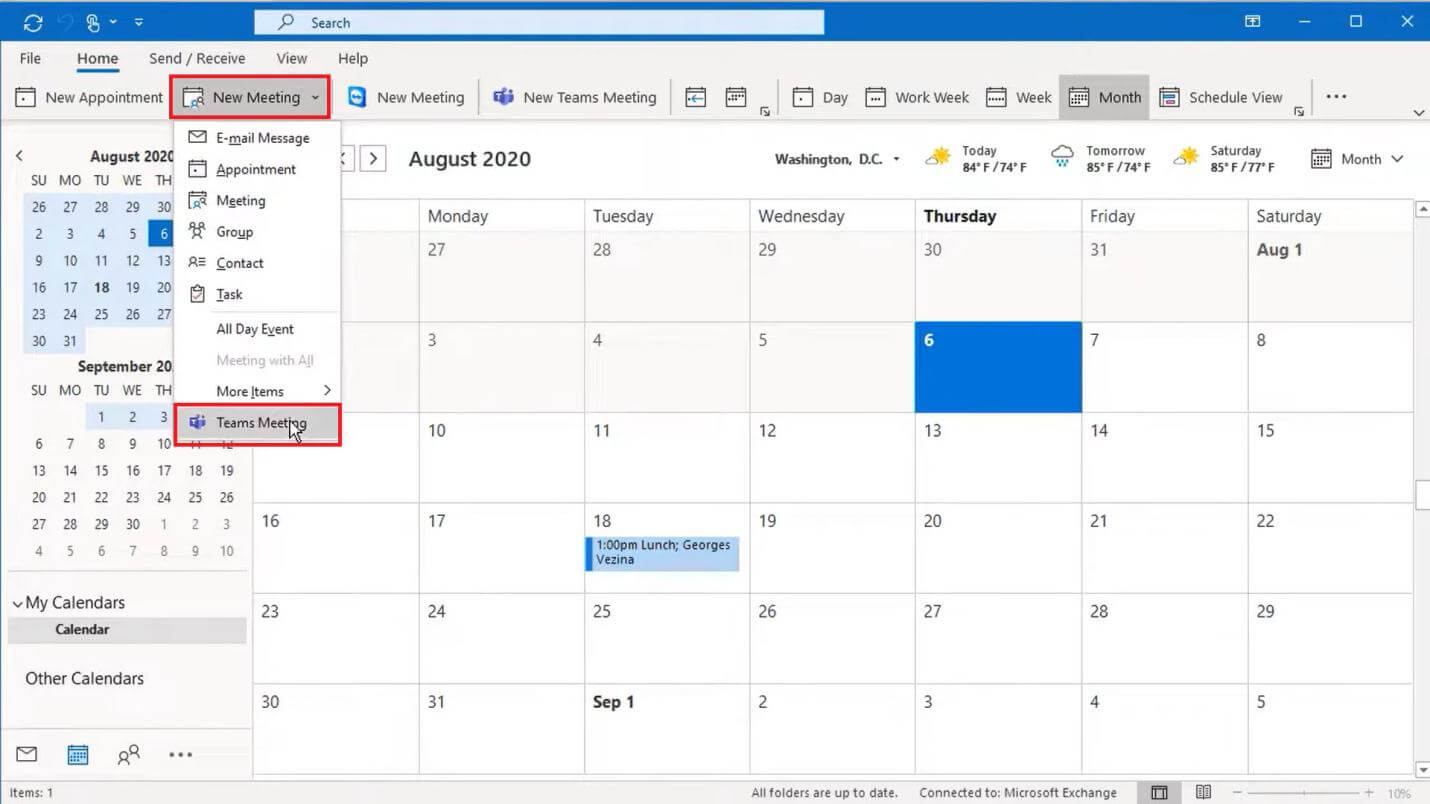The image displays a detailed screenshot of a digital calendar and email client interface. At the top, a blue background hosts several white icons, including a refresh symbol and a left-facing gray arrow. A finger icon is seen pressing a button. Left of center, there is a search function, and on the right-hand side, icons for minimize, maximize (square), and close (X) are visible.

Below the blue bar, on a white background, black text displays options such as "File," "Home," "Send," "Receive," "View," and "Help," with "Home" underlined in blue. A highlighted red section indicates a selection for "Meeting." Options for various email and calendar items include "Email Message," "Appointment," "Meeting," "Group," "Contact," "Task," "All-day Event," "More Items," and "Teams and Meetings." The white mouse cursor is positioned on the highlighted "Meeting" section.

Behind this interface, calendar views for August 2020 and September 2020 are visible. Additional details include options for "New Meeting," "New Teams Meeting," and various calendar views such as "Work Week," "Month," and "Schedule View." Information for August 2020 is displayed, including the weather forecast for Washington, D.C.: 

- Partly cloudy with a high of 84°F and low of 74°F for today.
- Thunderstorms with temperatures of 85°F and 74°F for tomorrow.
- Partly cloudy with 85°F and 77°F for Saturday.

The calendar highlights the last days of July (27th-31st) with August starting on a Saturday. September begins with the 1st through the 5th (Tuesday to Saturday). The 6th is prominently highlighted, and an event on the 18th, which is a Tuesday at 1 p.m., is noted as "Lunch with George's Vienna."